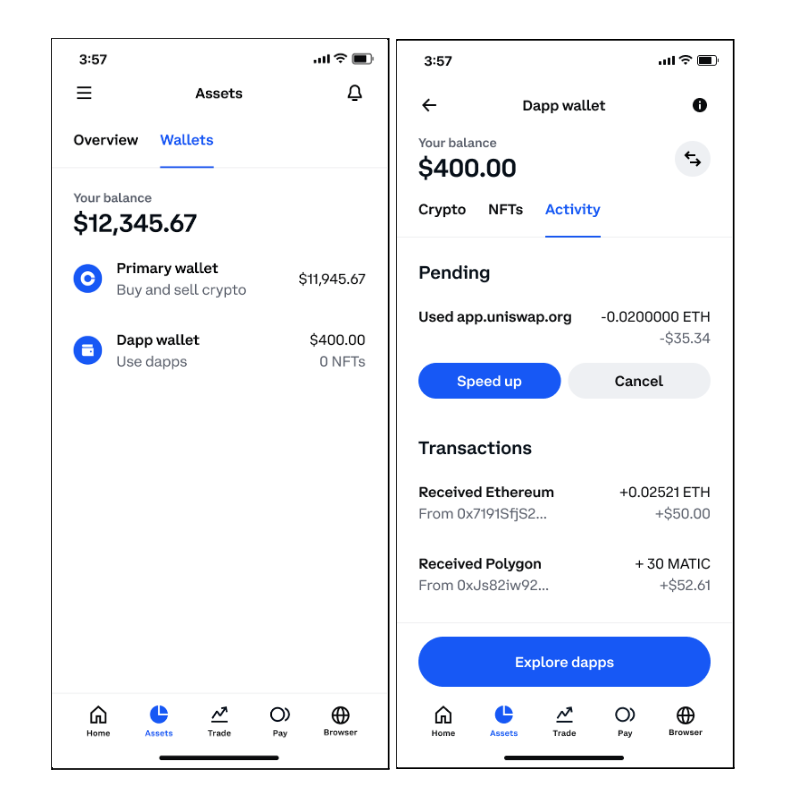The image features two screenshots displayed side by side, both in portrait mode, with the timestamp showing they were captured sequentially at 3:57 p.m. and 3:57 p.m. again. 

In the left screenshot, the top row reads "Assets," with "Overview" and "Wallets" listed underneath. "Wallets" is highlighted in blue and underlined. Below, the user's balance is displayed as $12,345.67. Further down, under "Primary Wallet," it shows "Buy and Sell Crypto" with a balance of $11,945.67. In the section labeled "DAP Wallet," a balance of $400 is listed, with zero NFTs, indicating a total balance comprising $11,945.67 in the primary wallet and $400 in the DAP wallet.

The right screenshot focuses on the "DAP Wallet," which again shows a balance of $400 and zero NFTs. The sections visible include "Crypto," "NFTs," and "Activity," with "Activity" underlined in blue, indicating it's the active section. It lists a pending transaction with the app "uni.swap.org," showing a negative balance of -0.0200000 ETH, equivalent to -$35.34. Additionally, there are two buttons at the bottom of this section: the left button in blue labeled "Speed Up" and the right button in gray labeled "Cancel."

Underneath the transaction details, there are records of received transactions, including received Polygon and Ethereum. Finally, at the very bottom, there's a button to "Explore DAPs."